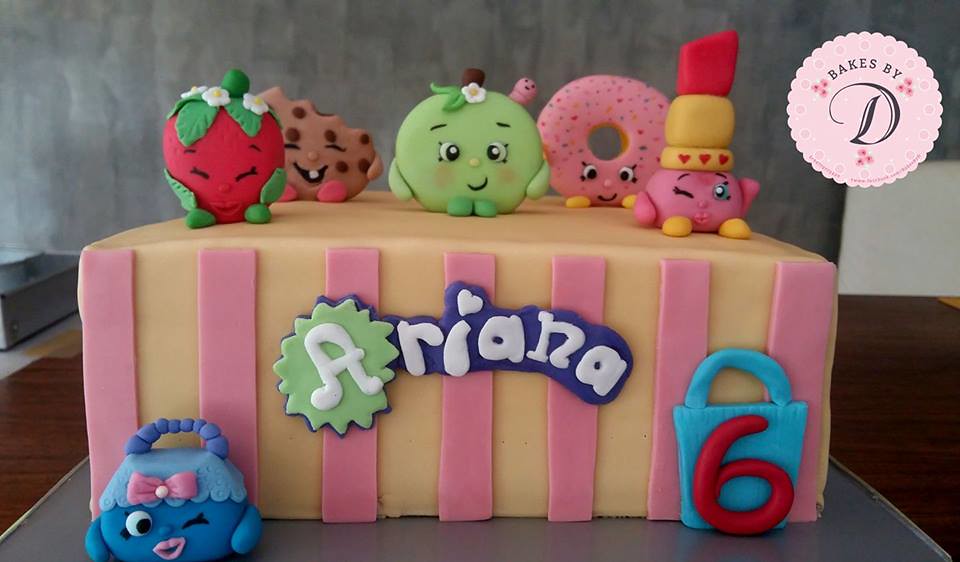This image showcases a meticulously crafted cake adorned with various intricate details. The front of the cake features striking pink and yellow stripes, with the base color being a soft tan. Centrally, the name "Ariana" is prominently displayed in white lettering, with a green star behind the initial "A" and the remaining letters in a purple hue. Additionally, there's a lock symbol bearing the number six on the right side of the cake, and to the left, a small, cartoon-like figurine.

The top of the cake is adorned with several edible figures, including a strawberry with a face, a cookie with a bite taken out of it, a green apple with a face, and a pink donut also sporting a face. There's also a whimsical figure with a face and a three-sectioned hat, resembling a bird with objects on its head. These figures appear to be made of liquid frosting or fondant clay. On one corner of the top, there is a circular emblem with the letters "FD," accompanied by the text "Bakes FD." The entire cake is designed to be fully edible, making it both a visual and culinary delight.